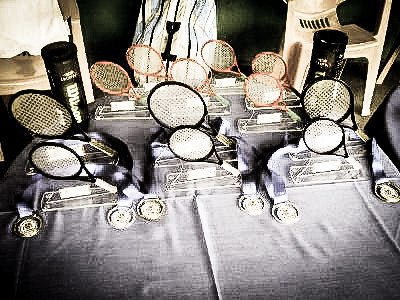The photo, though small and of poor quality, depicts a somewhat blurry and dark scene filled with various tennis-related objects. Central to the image are numerous tennis rackets of different sizes and materials, including black steel ones and smaller wooden ones, arranged in wire rack buggies with four wheels. These buggies are placed on a wooden floor, with a mix of rackets: to the left, there are two black ones, six red rackets are lined up across the back, and in the middle and right sections, there are more black rackets. Behind the buggies, there are plastic white chairs—one noticeably in the right top corner. Additionally, a blue and beige striped sports bag is centrally located in the photo. Next to this bag, on the left, there seems to be another chair or a table draped with a whitish-gray cloth. The brand "Wilson" can be faintly seen on the side of some of the objects, while the blurred circles near the front of the rackets could potentially be containers for tennis balls, adding to the confusion of the scene. The background also includes another piece of furniture, possibly draped with a cloth, which might suggest the setting is a garage or storage area.